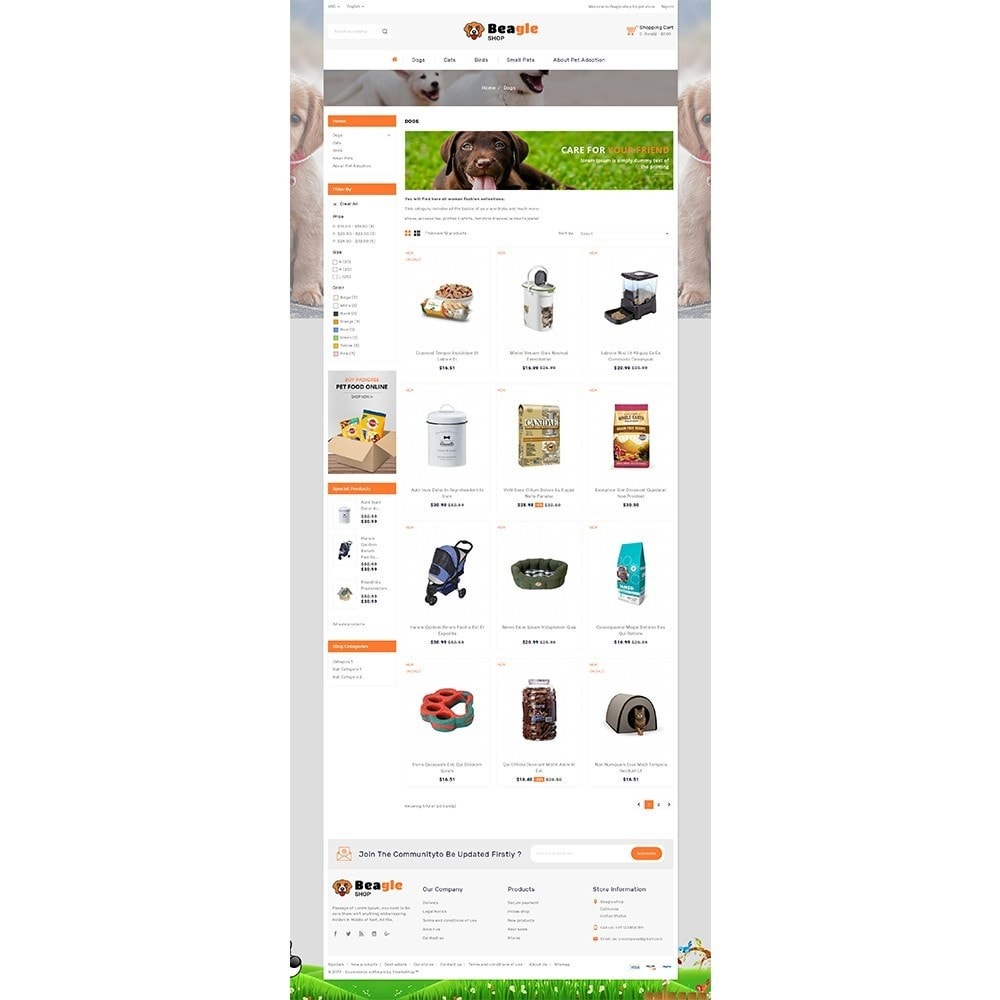This screenshot from the BeagleShop website offers a comprehensive overview of products designed for pet dog care. The site header features several tabs, likely for user sign-in and navigation, alongside the prominent BeagleShop banner. An illustrated Beagle logo is positioned on the left, with "Beagle" rendered in black for "B-E-A" and orange for "G-L-E." Beside the logo, a clickable orange shopping cart icon links to the user's cart.

On the far left of the banner sits a search bar, and below it is a navigation bar with tabs for Home, Dogs, Cats, Birds, Small Pets, and Pet Adoption. The left side of the page shows various filters for products, alongside an advertisement for Purina or a similar pet food brand. Other visible tabs include Sponsored Products and Recently Viewed Items, though the latter's text is slightly unclear.

The webpage background features playful illustrations of puppies, adding a charming touch to the layout. The main section displays 12 different products, each pertaining to dog care. At the bottom of the page, there is an invitation to "Join the Community" by subscribing to the newsletter.